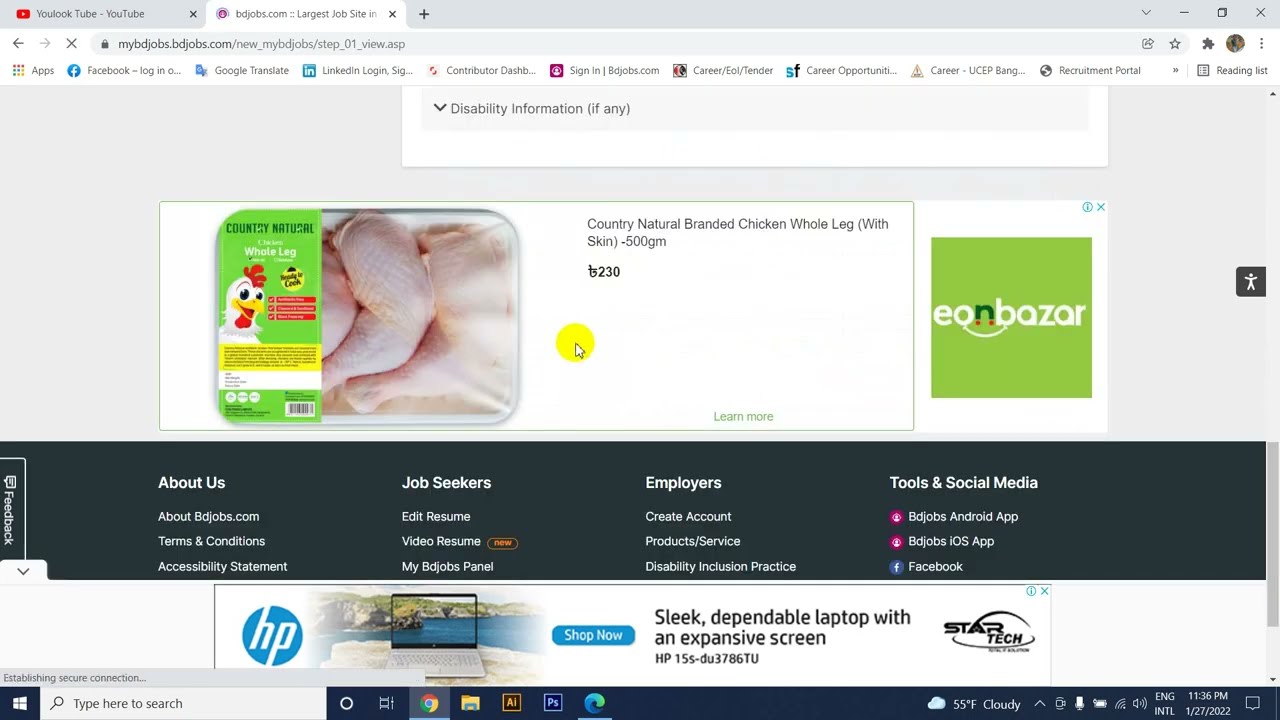Screenshot of a website browser showcasing various sections and detailed elements: 

The main portion of the webpage is divided into multiple sections. The top half displays a light gray background, followed by a dark gray rectangle with a green tinge, and below that, a white rectangle. At the very bottom of the webpage is a dark blue footer bar. The top of the light gray section features a white pane with a medium gray shadow cast behind it. There is a single light gray rectangle running almost the entire width of this pane. On the left side of this rectangle, a dark gray caret points downward next to the dark gray text that reads "disability information (if any)."

Beneath this white pane, separated by a small area of negative space, is a white rectangular advertisement. The left three-quarters of the advertisement are bordered by a thin light green line. On the right side of this bordered section, there is a green square with the words "Eon Bazaar." Most of the text is in white, except for the upper portion of the final "n," which is green, and the lower portion of the "B," which is red. A white cartoon smile extends from the bottom of the "O" to the bottom of the "B."

In the top right corner of the white pane, there is a blue eye icon with a blue circle around it, and even further to the right, there is a small blue "X." Within the green outline on the left side of the advertisement, there is a photograph of a package of chicken legs. To its right, there is a yellow circle with a white cursor outlined in black on top.